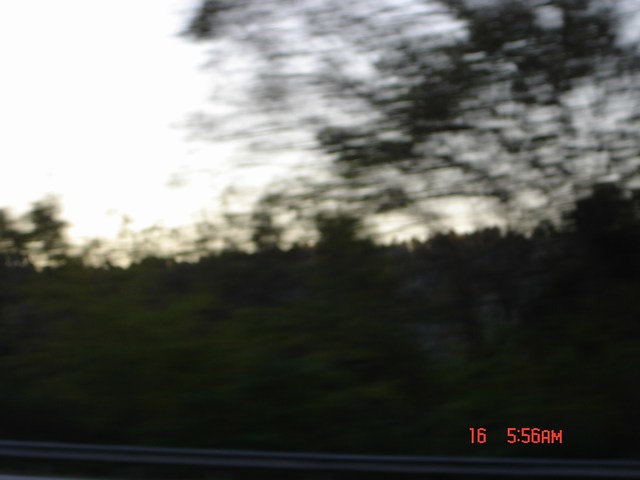This image is a horizontally rectangular, outdoor color photograph that appears to have been taken through the side window of a moving vehicle, likely at dawn. The photograph is somewhat blurry, enhancing the impression of high-speed motion. Dominating the background is a soft, light blue sky that transitions into shades of yellow and red near the horizon, suggesting an early morning sunrise. Dark green trees and dense foliage stretch across the horizon, with a particular larger tree that extends from just right of center to the right edge of the frame. The tree's leaves are sparse enough to allow glimpses of the glowing sky behind. In the foreground, a thin, black, metal-looking guardrail runs diagonally from the lower left to the lower right corner. The lower right corner of the image features red, digital-looking text displaying a timestamp: "16 5:56 a.m." Overall, the photograph captures a tranquil yet dynamic moment in nature, blurred by the movement of the vehicle.